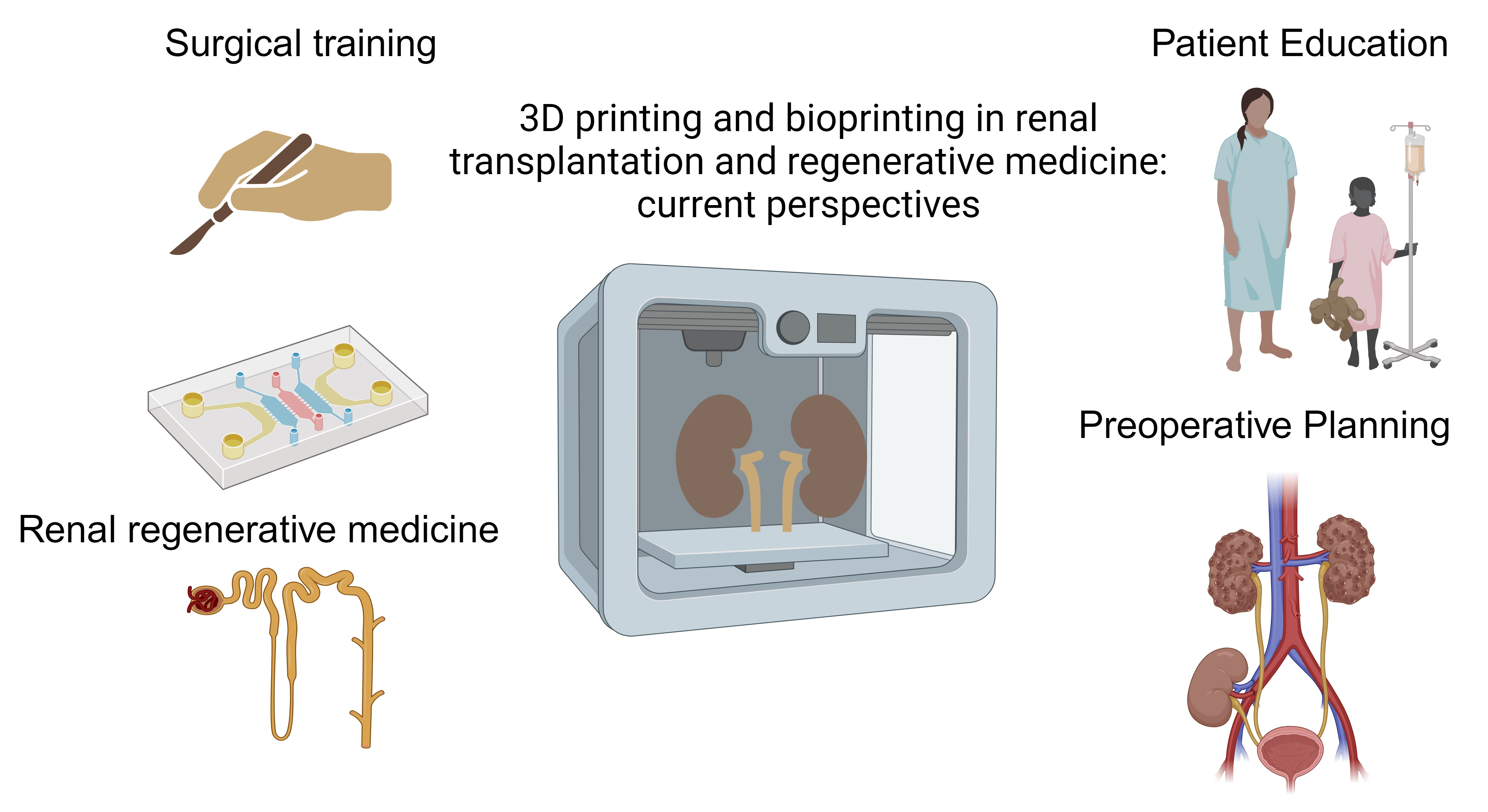This detailed image is a digital creation made up of six vector-style medical illustrations accompanied by descriptive text. 

Starting in the top left corner, black text reads "Surgical Training" above a beige-colored illustration of a hand holding a brown scalpel. Below this, a white rectangle features yellow, blue, and pink linear designs resembling a circuit board or electric circuits encased in glass. Further down, black text labeled "Renal Regenerative Medicine" is positioned above a tan, wiggly, organic structure resembling an intestine or organ with branching sections and a red veiny cluster at one end.

In the center of the image, bold black text states, "3D Printing and Bioprinting and Renal Transplantation and Regenerative Medicine: Current Perspectives." Directly beneath this text is a silver, six-sided figure, resembling a transparent 3D printer, containing structures that look like brown lungs or possibly kidneys.

Moving to the top right corner, small black text labeled "Patient Education" appears above an illustration of a woman and a small child in hospital gowns. The child is holding an IV stand with an IV bag. Below this, black text saying "Preoperative Planning" is positioned above illustrations of human body parts with prominently displayed red and blue veins, indicating a focus on vascular structures and preoperative anatomical planning.